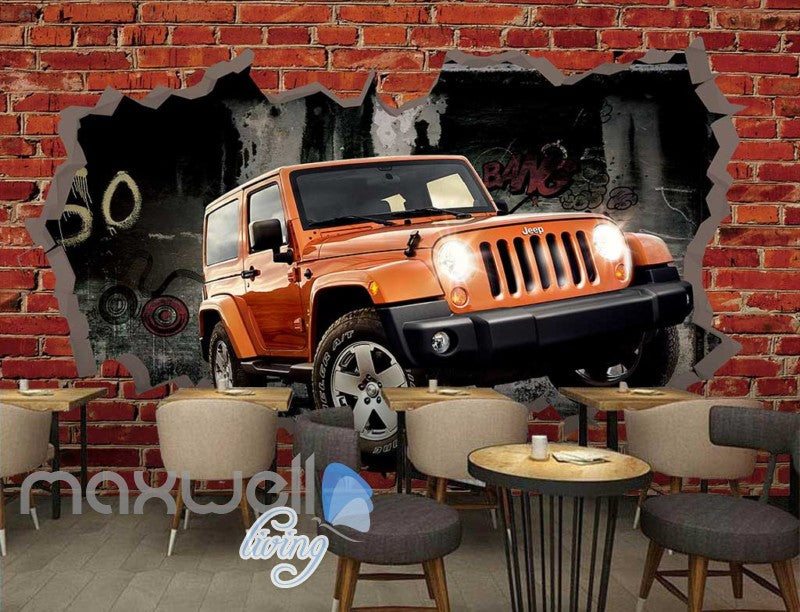The image depicts a detailed and vibrant mural on a red brick wall, featuring a highly realistic orange Jeep that appears to be breaking through the wall. The mural is masterfully crafted to create a 3D effect, complete with the Jeep's headlights turned on and the word "Jeep" prominently displayed on the front. The bricks around the mural are scattered and outlined in gray, enhancing the illusion of the Jeep bursting out. Below the mural, the setting indicates a café or restaurant environment, with several tables and chairs arranged neatly. On the tables, items like napkins and salt and pepper shakers can be seen, adding to the casual dining atmosphere. A circular table with two stools is positioned at the front right of the image, providing a cozy spot for patrons. The floor beneath is a gray color, complementing the overall brick motif. At the bottom left of the mural, the phrase "Maxwell Living" is inscribed, possibly indicating the name of the establishment or the artist's signature.